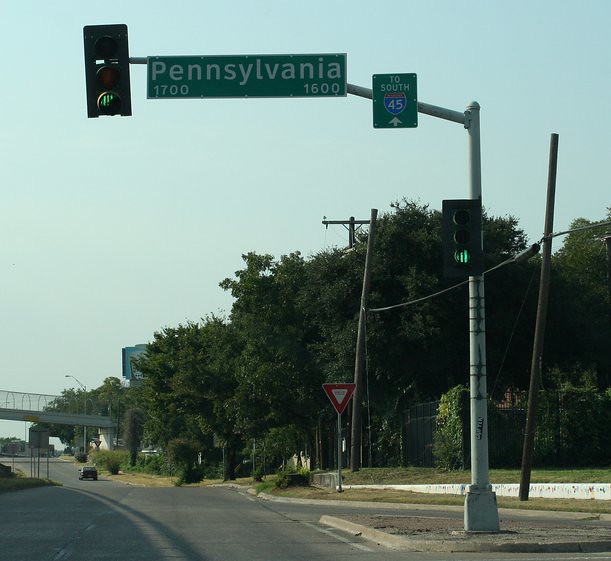This image depicts a roadway scene with a focus on a section of the road as it stretches into the distance, leading to a crossroads where vehicles can turn left or right. An overpass spans the crossroads. A lone, dark-colored passenger vehicle travels along the road. A traffic light stands prominently with a green sign indicating directions: Pennsylvania Avenue, with 1700 to the left, 1600 to the right, and South 45 marked on an interstate shield with a red top, blue bottom, and white numbers. Both the traffic signals, one on the pole and the other on an extended arm, display green lights. Trees line the right side of the image, and the overall ambiance suggests an overcast day with a gray-blue sky.